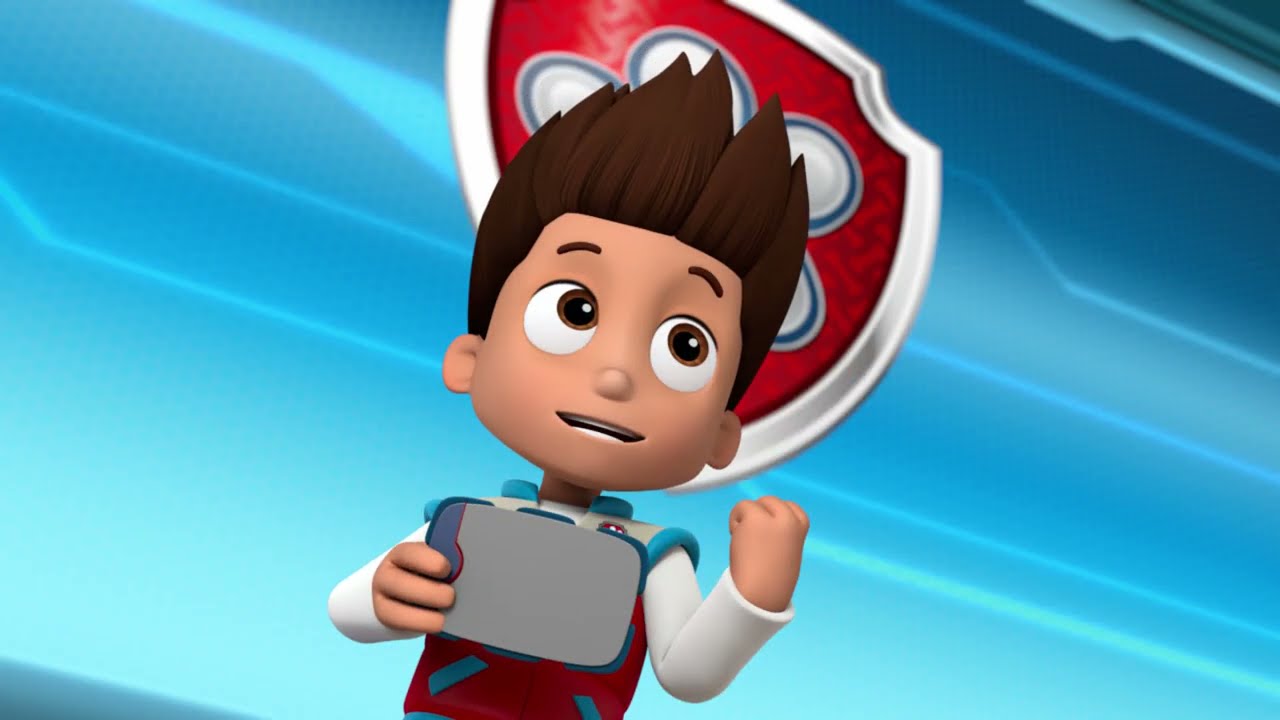The image depicts an animated, cartoon-like scene featuring a vibrant blue backdrop with cybernetic streaks running across different shades of blue, some illuminated and others darker, presented at a diagonal angle. At the center, a young boy with spiky, brown hair and large brown eyes gazes upward. He sports a red, white, and blue vest over a long-sleeved white shirt. His left arm is raised, with his fist clenched in a pumped, energetic motion, while his right hand holds a tablet. Positioned directly behind him is a shield with a white perimeter and a red face, featuring a blue-outlined paw print at its center, adding to the dynamic and spirited atmosphere of the scene.